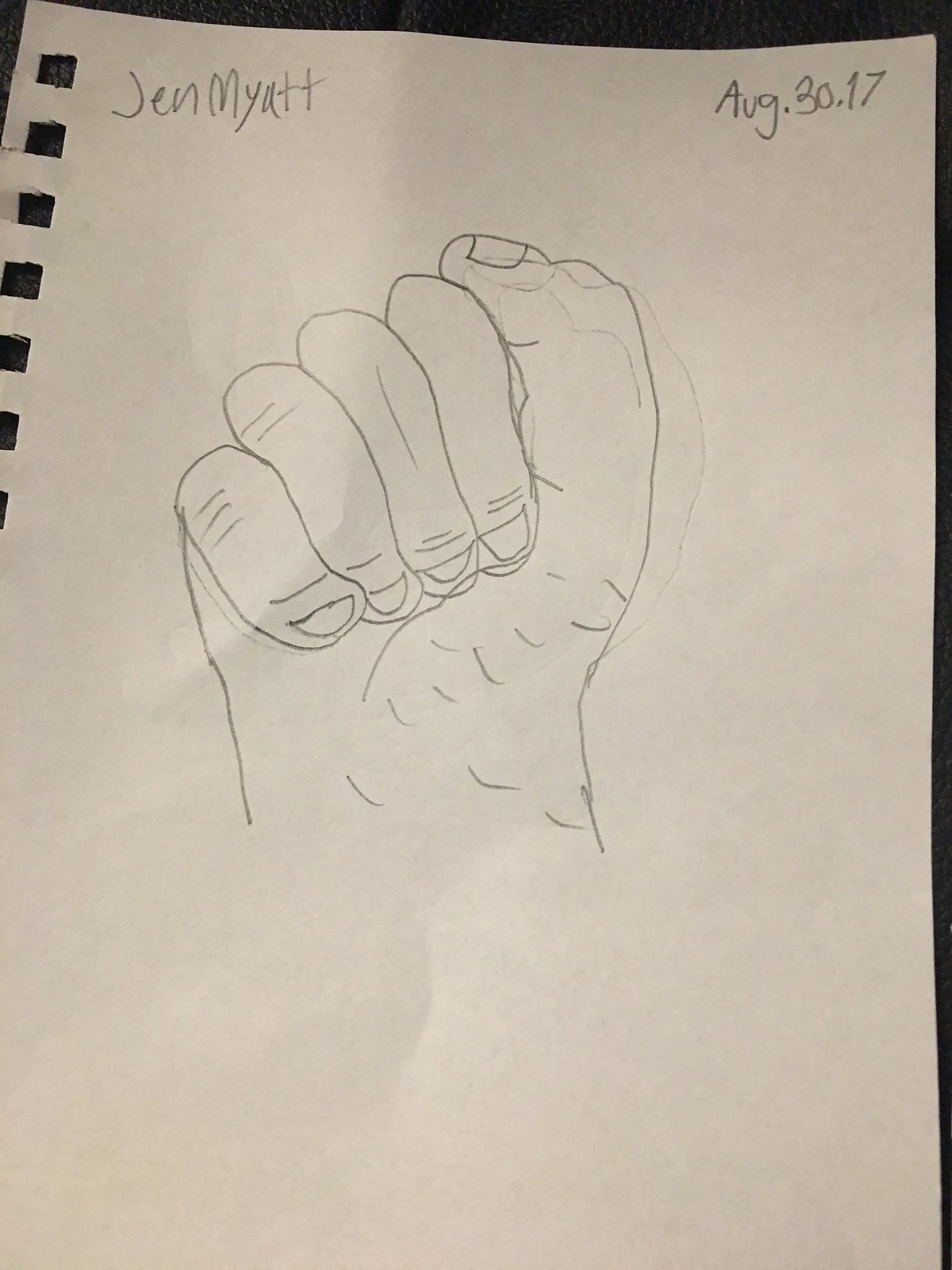The image features a roughly sketched drawing of a right hand, partially closed with the fingers touching the palm and the thumb resting on the side, revealing the fingernails. Notably, the nails have horizontal lines above them, and there are lines indicating knuckles and potential wrist hair. This sketch, rendered with pencil on a white piece of notebook paper—with the telltale spiral binding holes visible along one edge—includes some erasable marks around the thumb area. Authored by Jen Myatt, as inscribed at the upper left of the page, the drawing is dated August 30, 2017, as noted in the upper right corner. The background of the image is a plain black, emphasizing the starkness of the white paper.